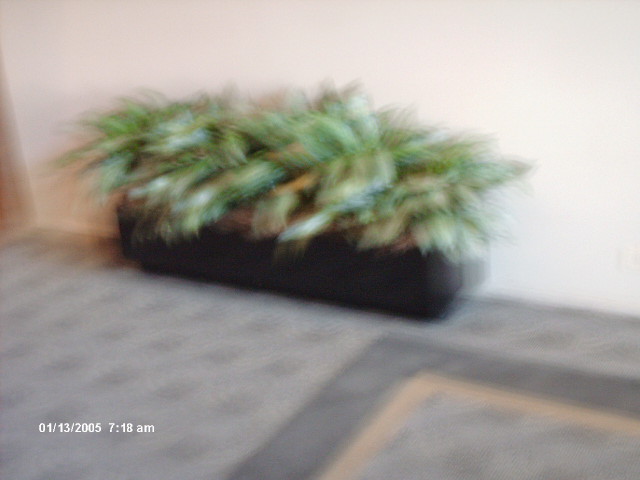In a somewhat blurry photograph taken on January 13, 2005, at 7:18 AM, a leafy container plant is prominently featured inside a building. The plant flaunts a lush array of dark green and white spiky leaves, tightly clustered together within a long, rectangular black planter. The planter rests against an off-white wall, placed atop a commercial-style rug that is primarily gray with dark blue designs. Brown dirt is visibly filling the planter, and shadows cast behind the foliage add depth to the image.